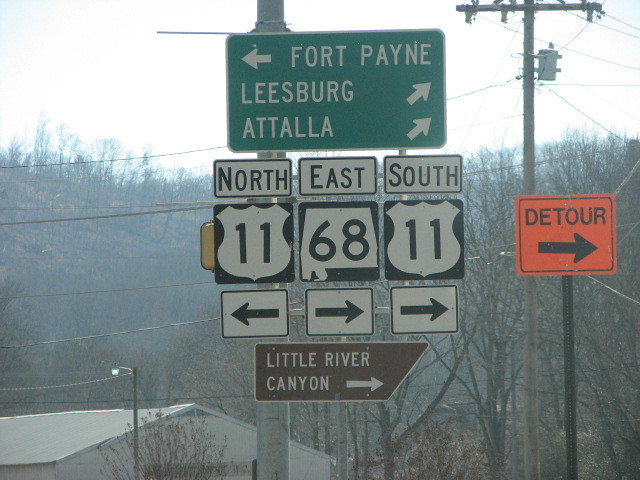At this small intersection, a multitude of signs directs travelers in various directions under a light, almost pastel sky. The backdrop features prominent hills adorned with sparse, leafless trees, hinting at late autumn or early winter. Electric poles and a web of power lines crisscross above, adding to the complex network of human infrastructure. 

A street light stands vigil near a large warehouse building, its industrial presence overshadowing the scene. To the right, a conspicuous orange detour sign indicates a change of route to the right. 

Above this, an array of road signs provides further guidance. At the top, a green sign outlined in white points left to Fort Payne and right to Leesburg and Atala. Below these, white signs with black lettering and borders indicate directions for North 11, East 68, and South 11. A distinctive brown sign with bold white letters guides visitors to the scenic Little River Canyon. The dense collection of signs at this intersection ensures no traveler is left without direction.